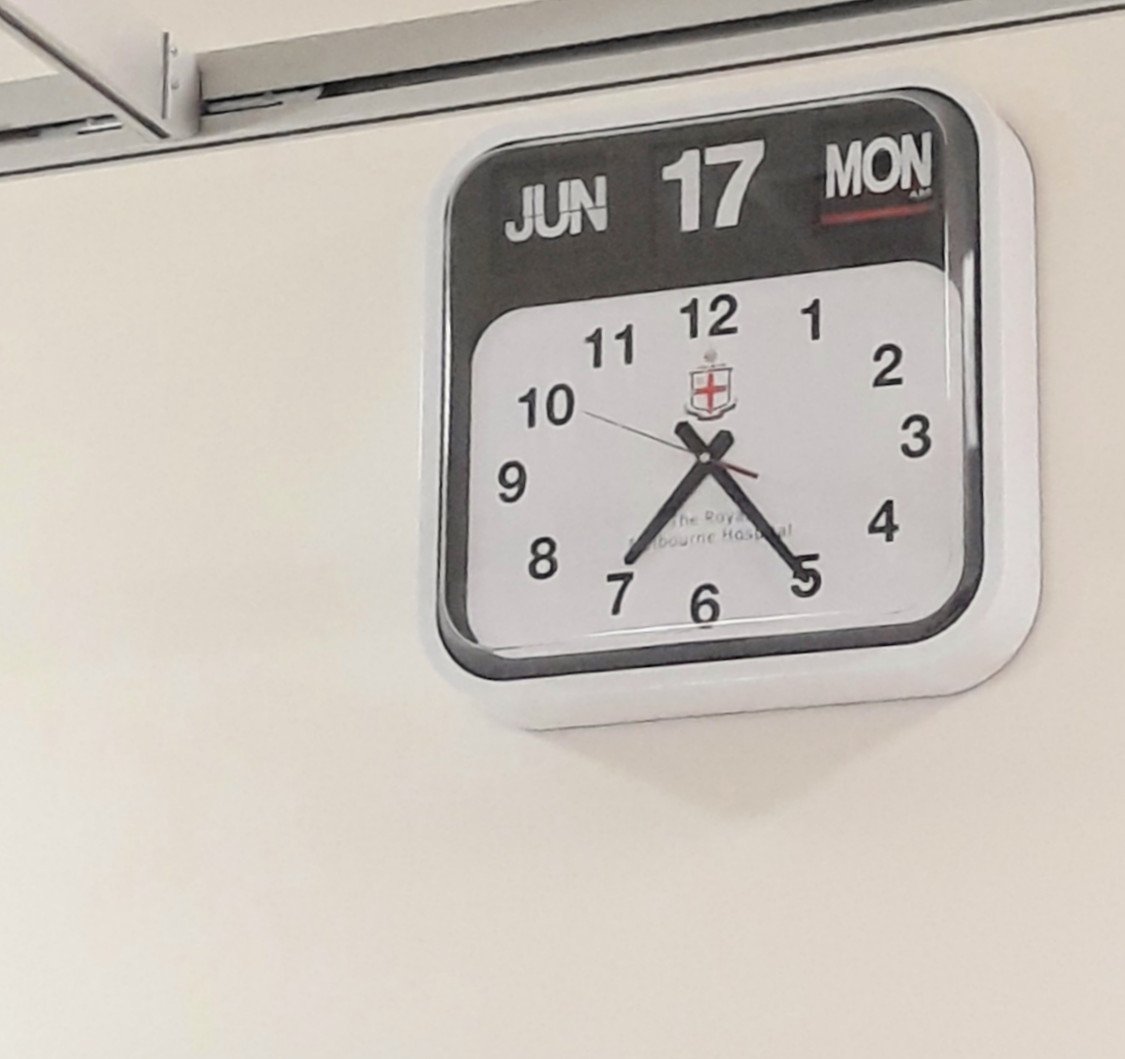This square, full-color photograph captures a wall-mounted clock prominently located in the upper right-hand corner. The plastic clock has a white, rounded-corner housing. The upper portion of the clock face features a black background displaying the date as "JUN 17 MON," with the number 17 noticeably large. Below the date display, the straightforward clock face shows the time 7:25, with plain numerals encircling the dial. A small, detailed crest with a red cross and a blue ribbon is positioned above the clock hands, below which the partially obscured text reads "The Royal Melbourne Hospital." The metallic pieces extend across the top and upper left corner of the frame, while the bottom background fades to pearl gray.